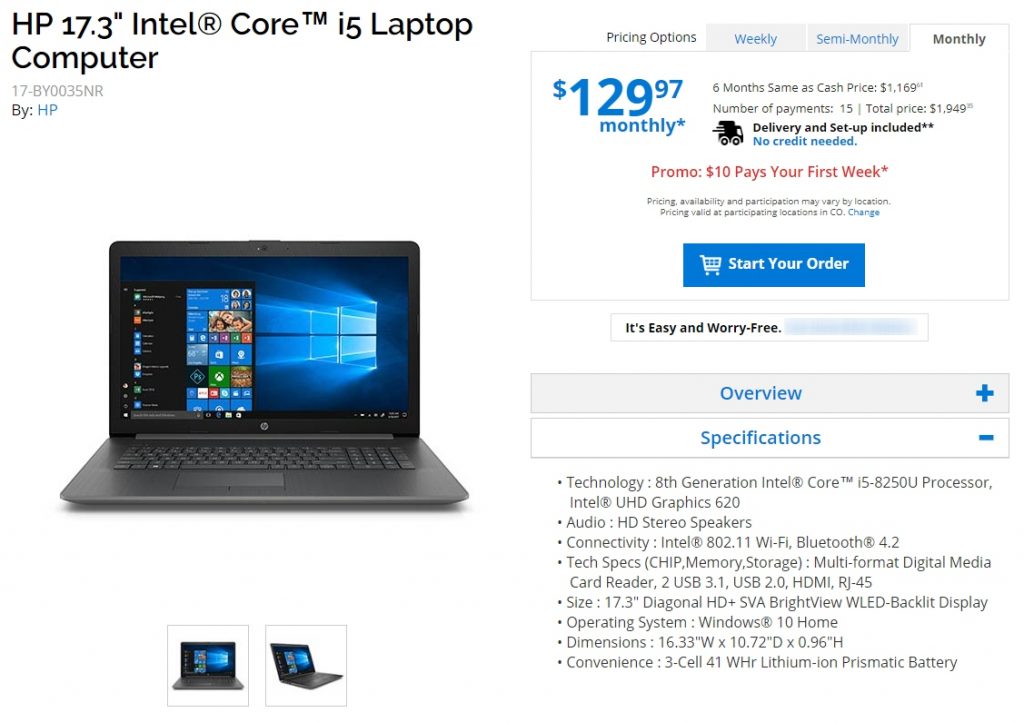**Detailed Description of the HP Core i5 Laptop Product Page**

This image depicts a product page screenshot for an HP Core i5 laptop computer, meticulously structured with vital information.

At the top left corner, the header prominently displays: "HP 17.3-inch Intel® Core™ i5 Laptop Computer." Directly beneath, a unique identifier "17-BY0035NR," follows, with the brand "HP" highlighted in blue text. The backdrop is predominantly white featuring black text.

Centrally positioned is a high-resolution image of the laptop, shown from a front view with the screen and keyboard visible, set against a white background and casting a subtle shadow. Below this primary image, two thumbnail previews offer different angles of the laptop, the default thumbnail showcasing the same frontal view, and the second one displaying the laptop at a slight angle in an open position.

On the right side, detailed product information is methodically laid out starting with the section titled "Pricing Options," accompanied by three selectable tabs: "Weekly," "Semi-Monthly," and "Monthly," with the "Monthly" tab currently active. The subsequent details include:

- **Price**: "$129.97 Monthly*" in blue text.
- **Terms**: "6 months same as cash price $1,169," "Number of payments 15," "Total price $1,949."
- **Delivery Info**: An icon of a truck in motion with "Delivery and Setup Included. No credit needed."

Below is a promotional notice in dark pink: "Promo: 10 days your first week." Following is a disclaimer in small black text: "Pricing Availability and Participation may vary by location. Pricing valid at participating locations in CO," with an adjacent blue link labeled "Change."

Further down, a prominent blue button bearing white text and a shopping cart icon invites users to "Start Your Order." Beneath this, a message reads, "It's easy and worry-free," although the continuation is obscured by a user-applied blur effect, all within a gray outlined box.

Lastly, two expandable accordion menus appear at the bottom:
- **Overview**: Collapsed and marked by a plus sign.
- **Specifications**: Expanded with a minus sign, revealing a detailed bulleted list of eight specific features and specifications regarding the laptop.

This comprehensive layout ensures potential buyers have access to all essential details, promoting an informed purchasing decision.